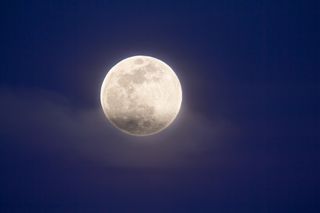This small, horizontally aligned rectangular image captures a full moon suspended in a dark blue sky that verges on black, evoking the onset of evening. The moon, perfectly round and slightly off-center towards the left, showcases a striking white or off-white surface accented with grayish-brown spots. Notably, a few wispy, feathery clouds hang just behind and below the moon, adding subtle texture to the scene. The moon's illumination lightly diffuses across the lower left and right areas of the image, creating a faint, murky light against the predominantly dark backdrop. This atmospheric picture emphasizes the moon's ethereal glow as it stands out amidst the twilight sky.